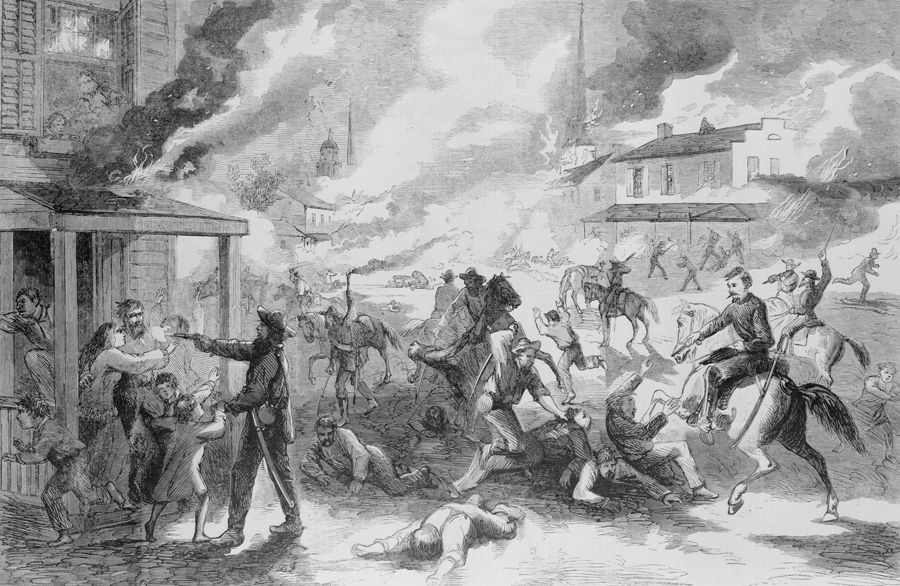This black-and-white illustration depicts a chaotic invasion of a small Western town, captured in fine pencil-style sketching with various shades of gray and black. On the left side of the image, a house with its upper story window belching smoke and flames hosts a dramatic scene: a family clutches each other in the entryway while a man in a hat, brandishing a gun, appears to have just fired at another man. Children are seen trying to intervene, clutching at the shooter to stop him. Men on horseback sweep through the right side of the image, dragging people around and violently beating and shooting them. The town's buildings, including a church with a prominent steeple, are ablaze, with light and dark gray smoke billowing into the sky. People, many wearing cowboy hats and overalls, run in panic through the streets amidst the mayhem, some lying dead or crawling on the ground. The scene is a vivid portrayal of the terror and destruction wrought upon the town.